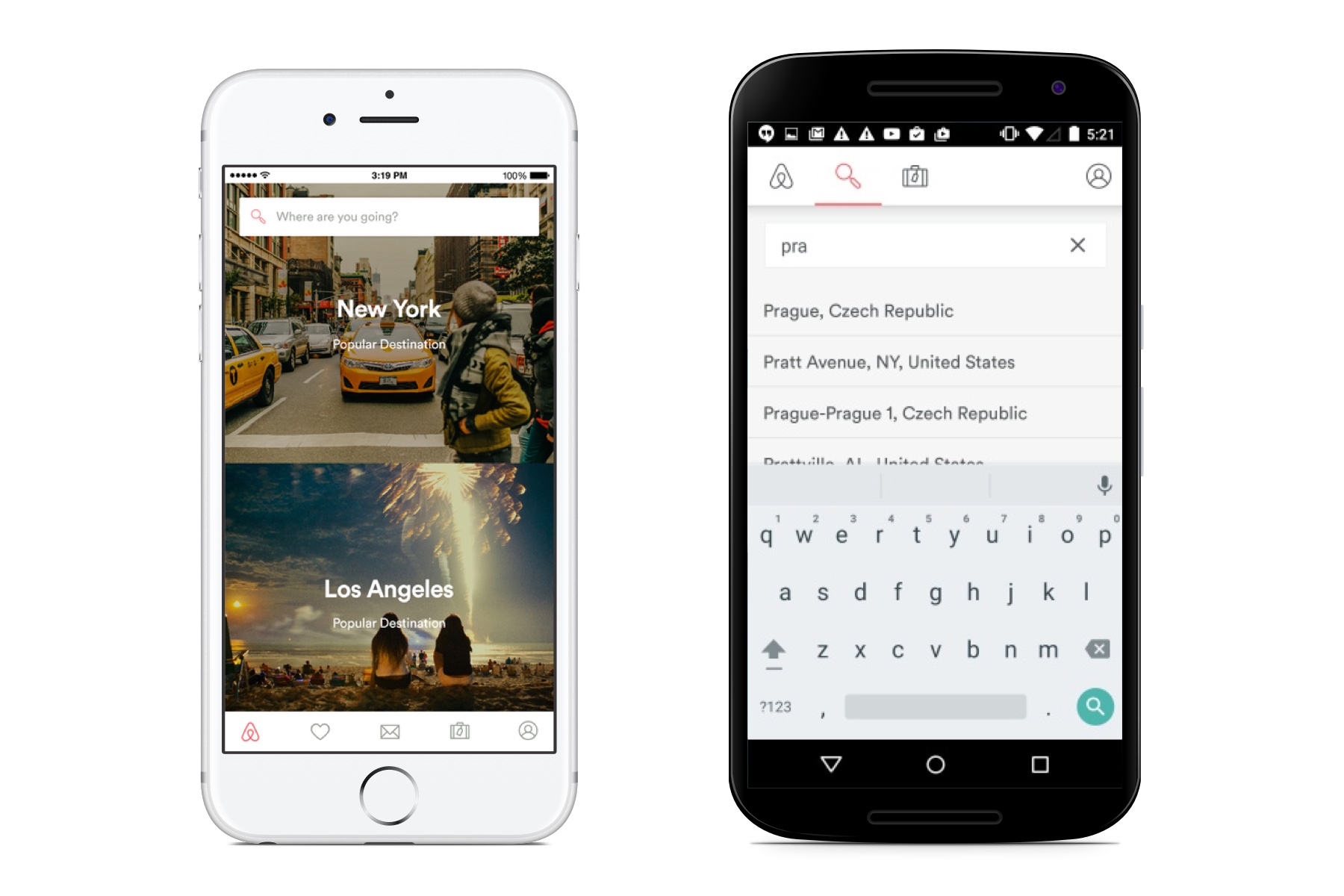In this image, there are two smartphones positioned side by side; an iPhone on the left and an Android phone on the right. The iPhone is white, and the Android phone is black. 

On the white iPhone's screen, there are two prominently displayed images. The first image features the text "New York" in bold, white, initial-capped font. Directly beneath this, in a smaller and lighter white font, are the words "Popular Destinations." The second image shows the text "Los Angeles," also in bold, white, initial-capped font, with "Popular Destinations" written below in a similarly smaller and lighter white font. This layout suggests that the iPhone is displaying a webpage related to travel and popular destinations.

At the top of the iPhone screen, a search bar is visible with a magnifying glass icon outlined in red. Inside the search bar, in a light gray font, the text reads, "Where are you going?" indicating that users can tap to type their travel destinations.

At the bottom of the iPhone screen, there are three icons: the red Airbnb logo, a heart icon trimmed in gray representing the 'favorites' feature, and a gray-trimmed envelope icon indicating the option to share content. These icons suggest functionality related to browsing, saving, and sharing travel destinations and accommodations.